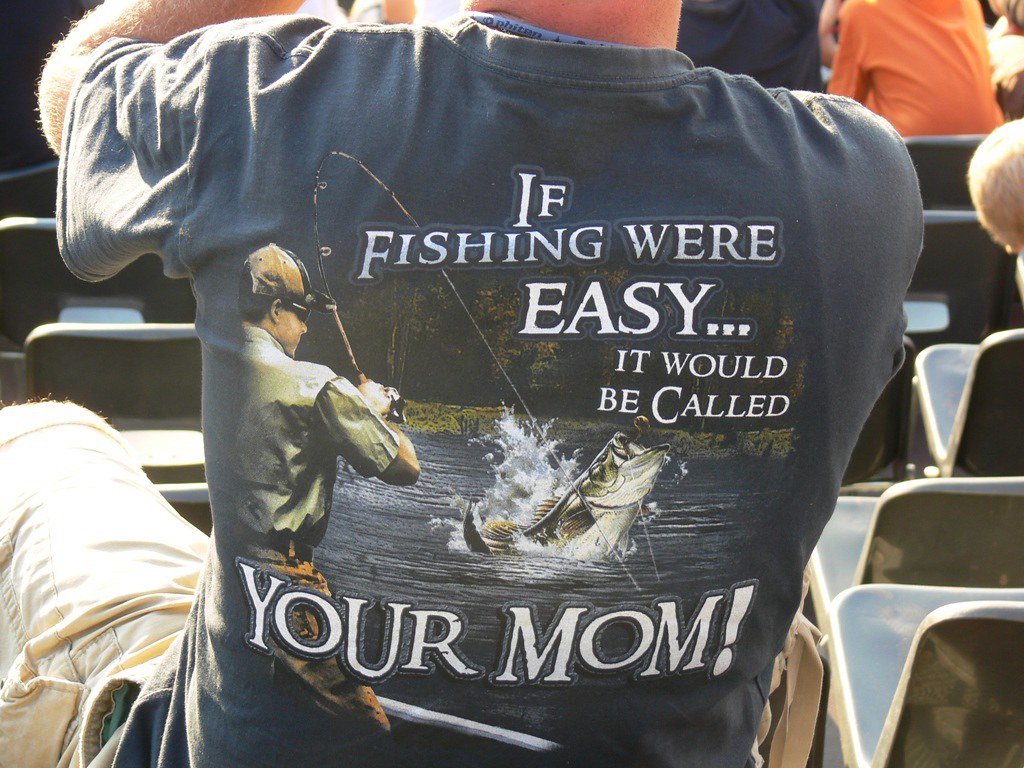The photograph is a close-up shot, depicting a man from the back, seated in a stadium amidst a crowd, possibly attending a baseball game or another event. The man is wearing tan cargo shorts and a dark blue t-shirt. The t-shirt features a large, detailed graphic of an angler wrangling a bass emerging from a stream, alongside a humorous, slightly provocative text in white that reads, "If fishing were easy, it would be called your mom." In the background, partially visible are the heads and backs of a few other spectators, including a little boy with blonde hair and individuals in navy blue and orange shirts. The image captures a slice of the stadium atmosphere with a focus on the man's distinctive and eye-catching t-shirt.